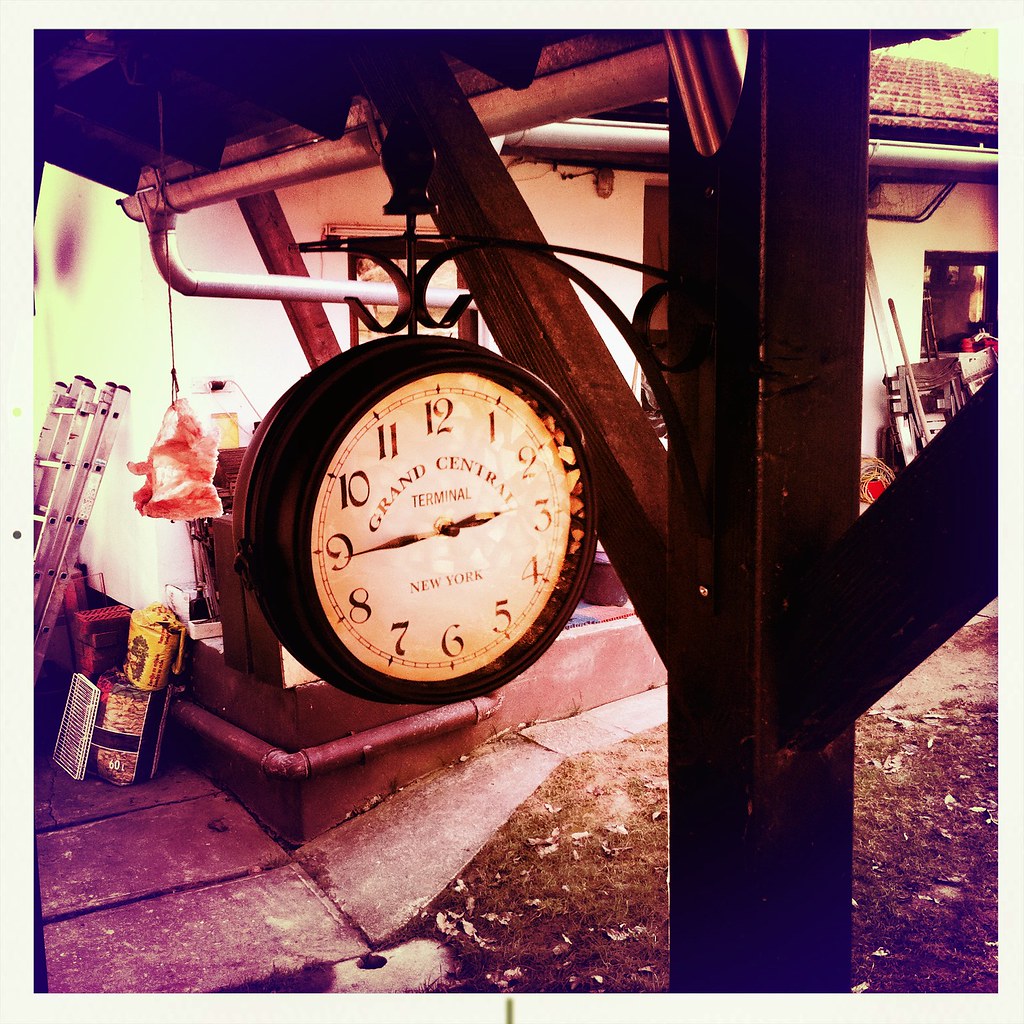This photograph captures a backyard scene bathed in an almost reddish hue, giving it an old-style, nostalgic feel reminiscent of a 70s or 80s photograph. The focal point of the image is a retro, circular clock hanging from a Y-shaped wooden post, displaying the words "Grand Central Terminal, New York"—an evident design element rather than its actual location. The clock's hands point to 9 and 3, emphasizing its vintage look with black numerals. In the background, we see a house with various miscellaneous items scattered around, including a ladder leaning against the side of the home, some bags, and different objects. Leaves are scattered across the lawn, and cement blocks sit at the bottom left corner. Tubes and pipe fittings crisscross the upper part of the image, adding to the cluttered yet quaint ambiance of the backyard.